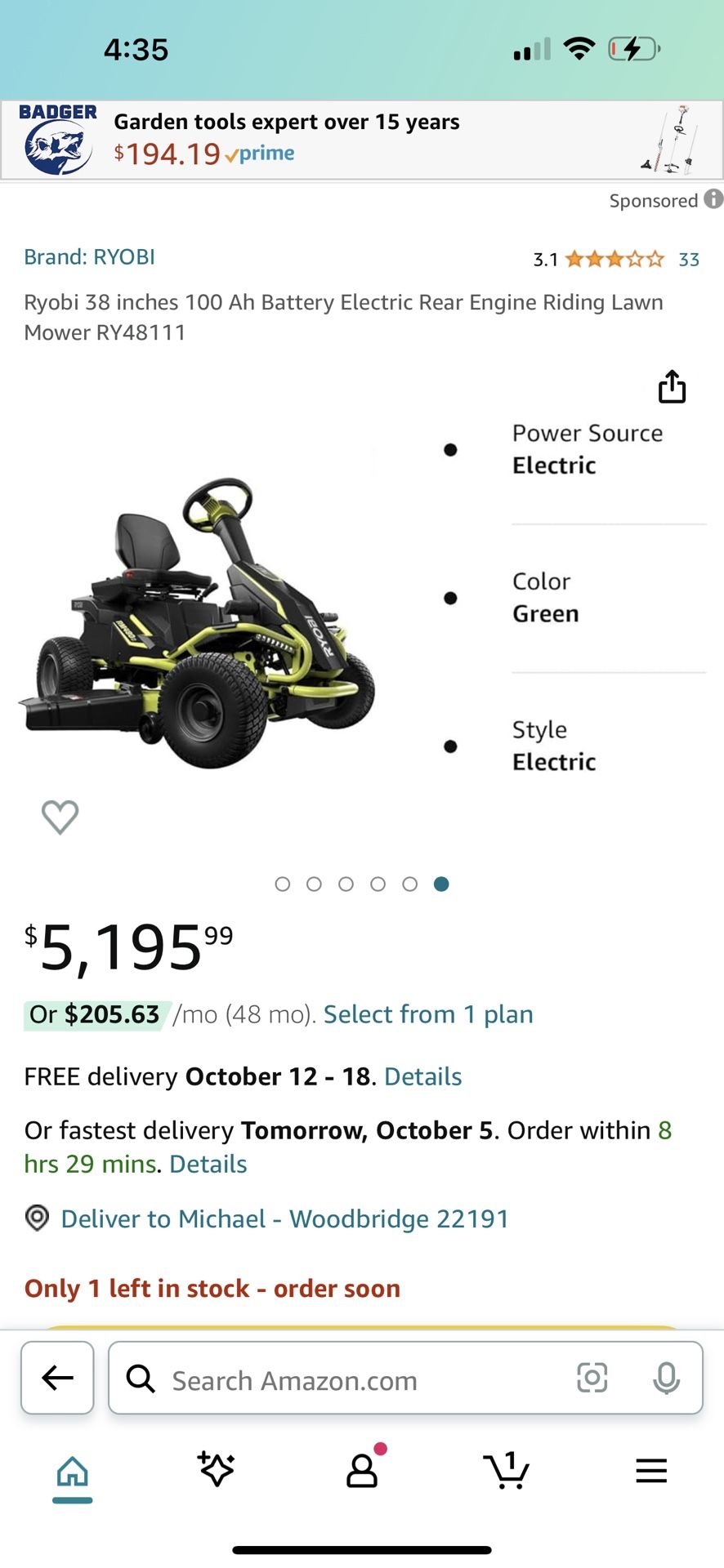The image depicts a webpage displayed on a smartphone, evident from the standard mobile status bar at the top, which indicates that the battery is nearly depleted but currently charging. The phone shows two bars for cellular signal strength while the Wi-Fi connection is fully active. The webpage belongs to a company named "Badger," identifiable by the company logo featuring an image of a badger, situated below the website header. The site appears to specialize in garden tools, boasting over 15 years of expertise.

The user is viewing a detailed product page for an electric lawnmower, which resembles a tractor but is distinct from a traditional push mower. The listed price of the mower is $5,195.99, with an alternative financing option of $205 per month over 48 months. A promotional offer guarantees free delivery if purchased between October 12th and 18th, with the fastest delivery option available by tomorrow—a date indicated to be October 5th, suggesting the current browsing date is October 4th.

An address field shows the delivery location set for "Michael on Woodbridge," hinting at the user’s saved or preferred delivery address. This transaction is being processed through the Amazon platform, as evidenced by the Amazon branding on the page. The status suggests that the user is considering the purchase, but has not yet completed it, though a mention of a balance of $194.19 associated with Amazon Prime raises questions about whether it is a refund or an account balance.